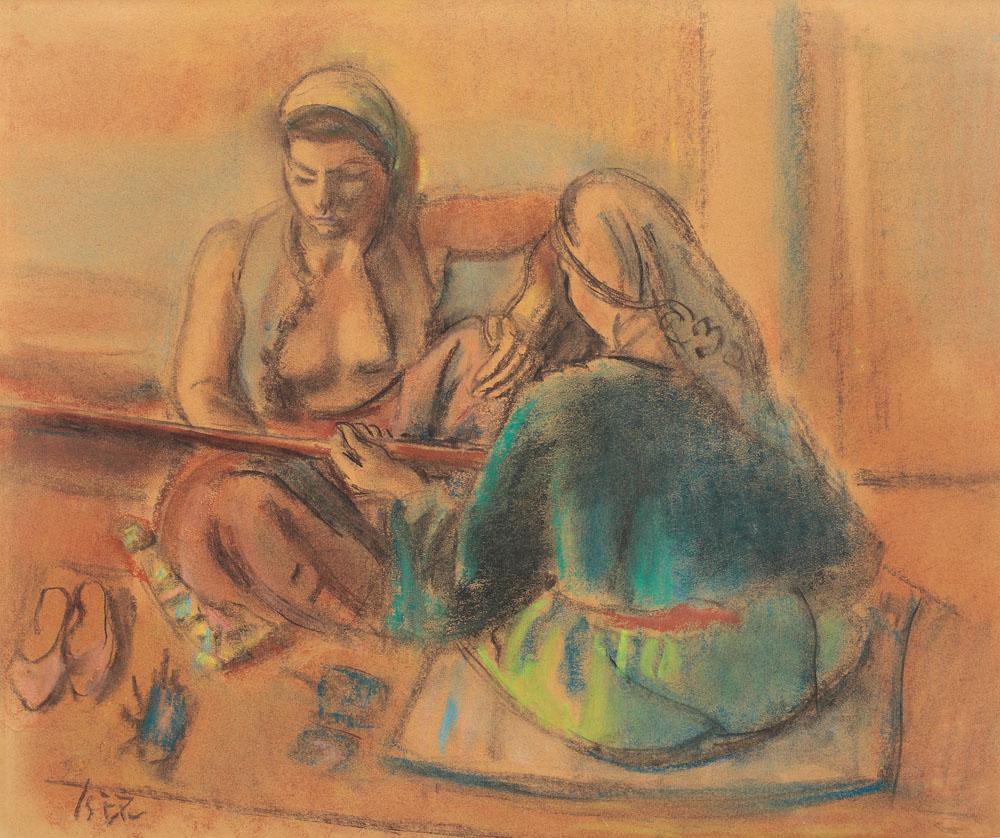The painting depicts two women sitting on the floor in a somber, muted setting. Both women wear head scarves, with the woman on the right dressed in a blue long-sleeve gown and green pants, while the woman on the left is clothed in a light tan, possibly uniform-like outfit with pink pants and a vest. The central focus of the artwork is on a brown wooden rod or instrument that both women are holding and looking down upon intently. They sit on a cushion or carpet, surrounded by sandals and various indistinct objects on the floor that resemble bugs. The scene appears somewhat blurry and lacks fine detail, with a signature in the lower left corner that is not clearly legible. The background features hues of light pink, red, and blue, contributing to the overall somber and muted tone of the composition.